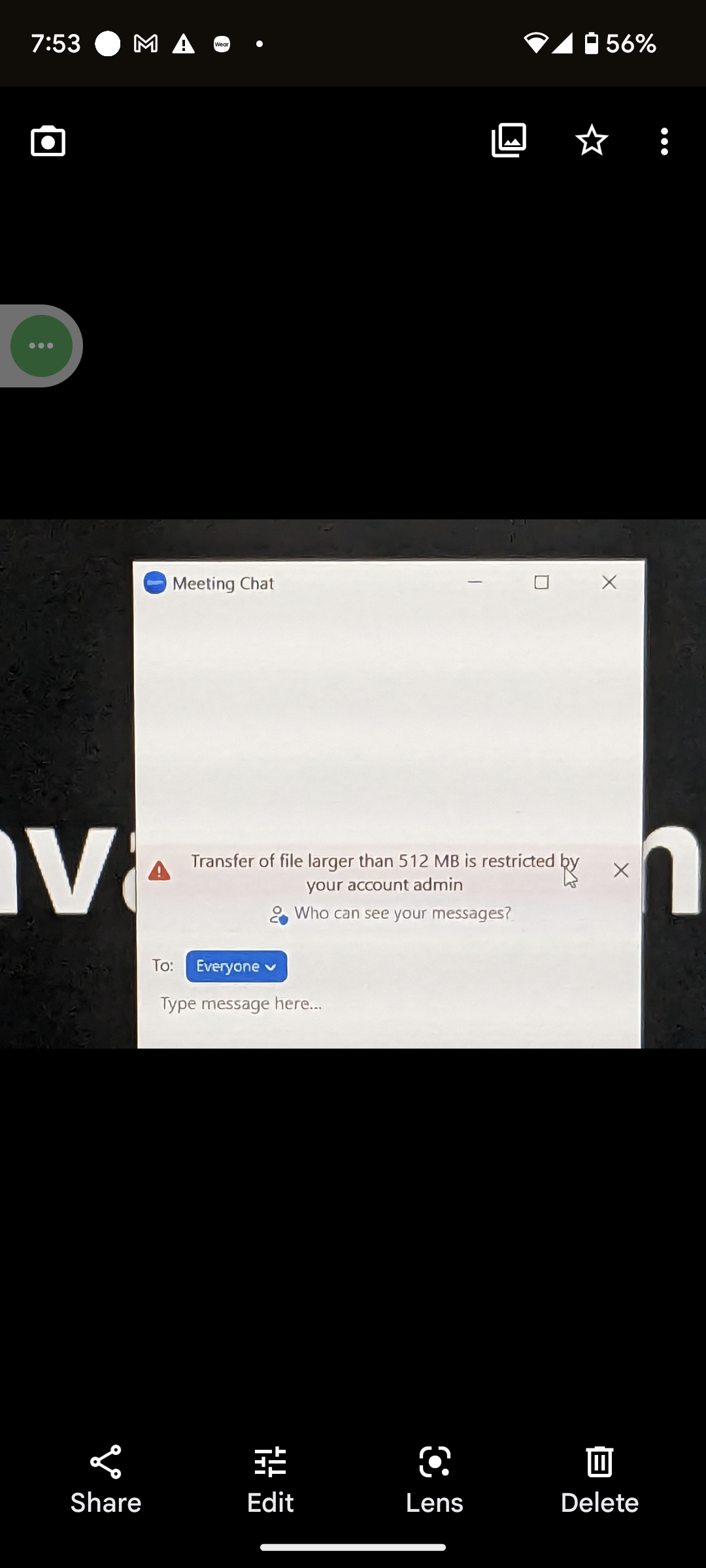### Caption:

A detailed screenshot of a phone screen displaying a black background with various icons, text, and notifications:

- **Top of the Screen**:
  - **Left to Right**: White text indicating the time "7:53".
  - Next to it is a large white dot.
  - Following that is an icon "DM" for Gmail.
  - A white triangle with a black exclamation mark warning icon.
  - A white circle containing black, illegible text.
  - Another white dot to its right.
  - On the far right, a Wi-Fi signal icon showing full strength with five bars.
  - Next to it, a battery icon indicating 56% charge.

- **Middle Section**:
  - **Left Side**: A camera icon.
  - **Far Right**: Two overlapping square icons resembling photo gallery symbols.
  - To the right of that, a white outline star.
  - To the right of the star, three vertically aligned white dots.

- **Left Side**: Google Assistant tab is visible mid-screen, with a smaller green dot accompanied by three horizontal white dots.

- **Bottom Section**:
  - A prominent white pop-up takes center stage.
  - **Top Left of the Pop-up**: A blue circle with illegible white text.
  - To the right of the blue circle, the text "Meeting chat".
  - Below that is a blank text input box.
  - Further down to the left, a red triangle with a white exclamation mark and text reading "Transfer a file larger than 512 MB as restricted by your account admin."
  - To the right of this warning, a human icon with a blue dot that says "Who can see your messages."
  - To the left of this text is "To: Everyone" in white on a blue rectangle.
  - At the base of the pop-up, a prompt "Type message here".
  - **Bottom Row**: Action buttons labeled:
    - "Share" with a share icon above it.
    - "Edit" with an edit icon above.
    - "Lens" with a lens icon.
    - "Delete" with a trash can icon above it. 

The image captures the multitasking and communication capabilities of the phone, with visual indicators for messages, file transfer restrictions, and bottom navigation options.